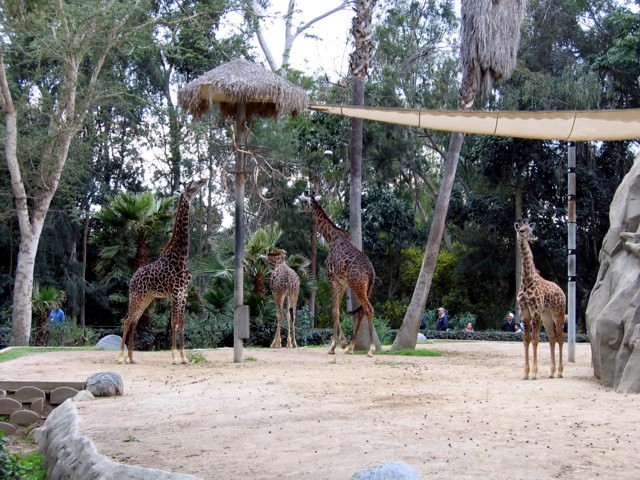The image is a color photograph, taken in a landscape orientation, depicting a zoo exhibit featuring at least four giraffes—three of which appear to be adults, with one smaller in size. The giraffes stand on a levelled, sandy terrain that resembles beach sand, situated on a raised platform supported by visible stones in the bottom left corner. The sandy area is not enclosed by any visible fences, suggesting an open, zoo-like habitat. Central to the image is a vertical metal pole implanted into the sand, topped with an umbrella-shaped structure covered in hay or straw, likely providing the giraffes with both food and shelter from rain. This structure has straw protruding from underneath the umbrella. In the background, lush greenery with various trees and shrubs frames the scene, with an overexposed white sky visible through the foliage gaps. Visible walkways and visitors in the distance indicate this is a public exhibit designed for optimal viewing from multiple angles.